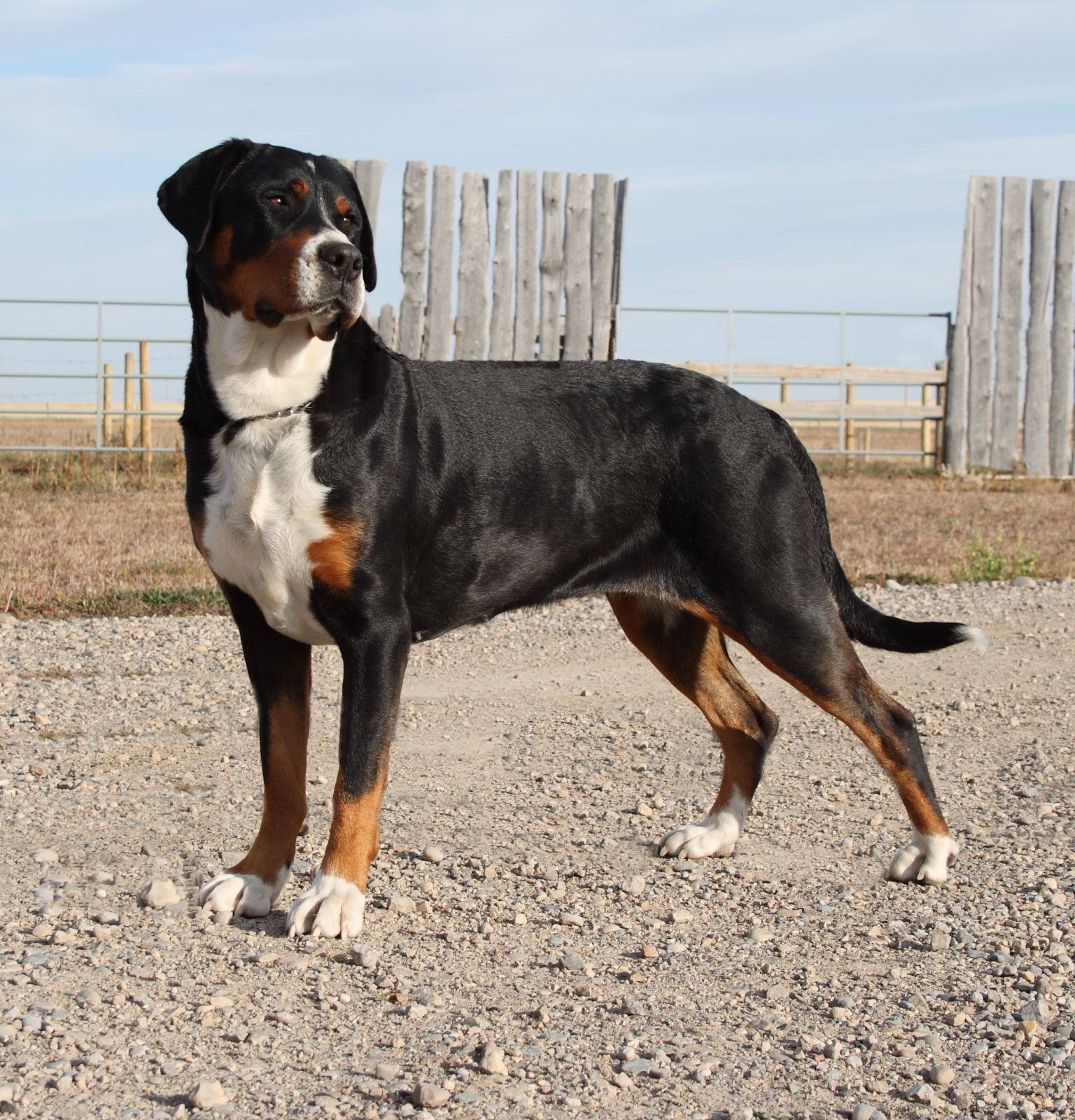This is a rectangular photograph, slightly taller than it is wide, capturing a mid-sized dog standing on a gravel path. The dog displays a striking tri-color coat predominantly black with distinctive white and brown markings. Its black coat is accented by a white chest and neck, a white line extending up the snout to the head, and brown tips on its legs, face, and a dot near the left leg. The snout is white with a black nose, and the expressive brown eyes gaze toward the right, counterbalancing its body, which faces left. Its ears are short and rounded. Above its black tail, a white tip stands out against the backdrop of a light blue sky filled with overcast clouds. The gravel path appears well-trodden, surrounded by a field of dead grass and an arrangement of both wooden and metallic fence posts. In the background, there is a metal gate and wooden struts, adding to the rustic ambiance.